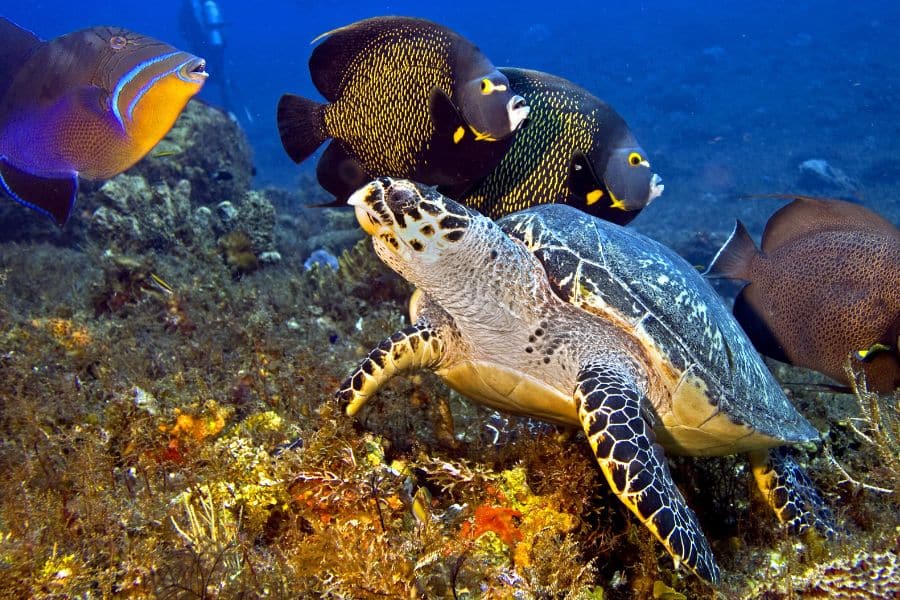This underwater scene captures a vivid portrayal of marine life against a backdrop of seagrass in hues of yellow and orange. In the foreground, a large sea turtle, identifiable by its black shell adorned with yellow markings and a distinct white neck and head accentuated with black patterns, is swimming from right to left. Just behind the turtle are two disc-shaped black fish, notable for their bright yellow spots and eyes, as well as white mouths. Further in the background and slightly to the left of these two fish, a brown fish with a similar shape can be seen. Behind these creatures, a distinctive beige fish, with neon blue horizontal stripes over its mouth and a bright yellow underbelly, is also prominent. Hazy in the distant background, a diver equipped with an oxygen tank can be observed, adding a sense of scale and human presence to this vibrant aquatic tableau. The entire scene is bathed in light, which appears to emanate from just in front or below the sea turtle, illuminating the various shades and patterns of the underwater flora and fauna.